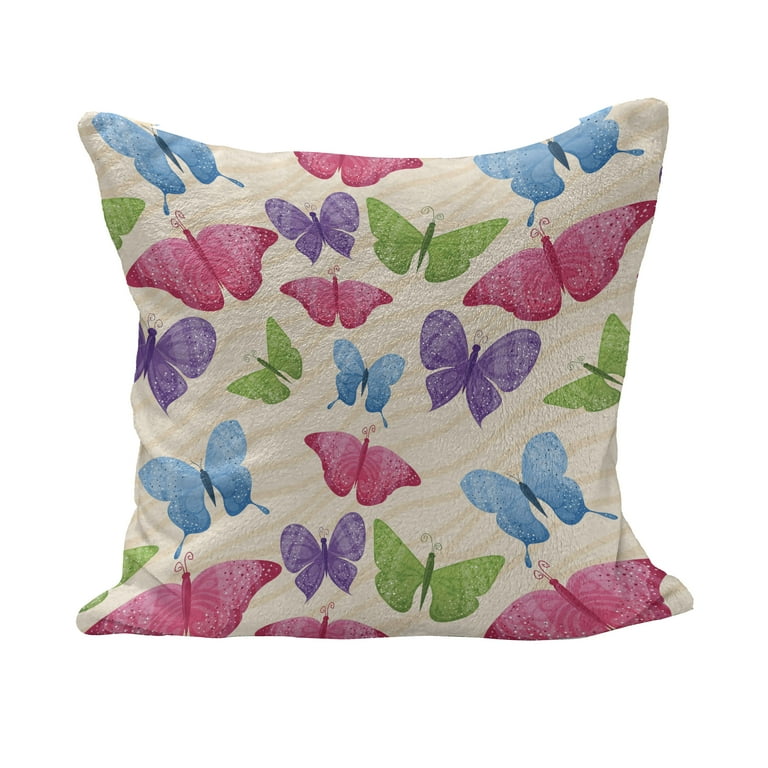The image showcases a square throw pillow with slightly tapered corners, giving it an elongated appearance. The pillow features a light beige background adorned with beige stripes, creating a subtle textured effect. Scattered across the pillow are assorted colorful butterflies in hues of green, blue, pink, deep purple, and fuchsia. Each butterfly is depicted in flight, with wings open wide, and their bodies and antennae match their wing colors. Some butterflies have spots and vary in size, contributing to a dynamic, unstructured pattern. Notably, some butterflies are cut off at the pillow’s edges, enhancing the notion of movement. The top of the pillow reveals a cream-colored zipper closure, with the tab clearly visible, implying practicality alongside aesthetic appeal. There is no text on the image, just a delightful, soft-looking pillow that emphasizes the vibrant, whimsical butterflies against a neutral backdrop.